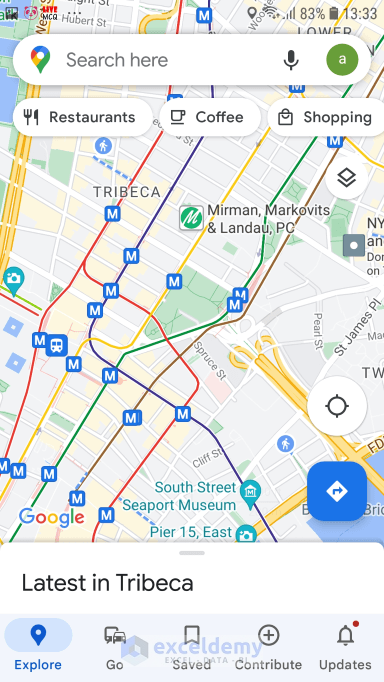This screenshot from the Google Maps app on a smartphone depicts a detailed map of Tribeca in lower Manhattan. The time displayed in the upper right corner is 13:33, indicating a 24-hour clock format, and the battery is charged to 83%. The map fills the entire screen, with a white, rounded-corner Google search bar at the top that includes categories for "Restaurants," "Coffee," and "Shopping," each enclosed in small, rounded rectangles.

Towards the lower section of the screen, the phrase "Latest in Tribeca" is visible, hinting at recent updates or points of interest in the area. In green text near the bottom, "South Street Seaport Museum" is listed as a notable location. The word "Tribeca" is prominently displayed towards the upper part of the map. Blue lines indicate bus routes, clearly marked with blue squares containing the letter "M." The map does not highlight numerous other points of interest, focusing instead on the broader layout and essential features of the Tribeca area.